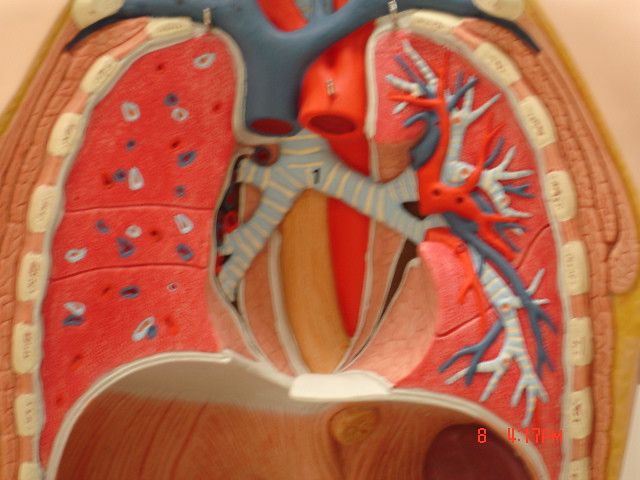The image depicts a detailed 3D model of a cross-section of a human torso, showcasing various internal structures. The primary focus is on the intricate display of arteries and veins, with prominent blue and red hues representing different types of blood vessels. The model highlights the lungs, which are primarily red, with blue and light blue circles indicative of additional anatomical features. Despite the detailed musculature and connective tissues, the actual heart is not present, creating an empty space where it should be. The model is set against a wood grain background and includes tissue and fat depictions to emphasize its instructional nature, likely as educational material. Small details like blue and yellow striped veins, as well as etched spots in blue and white, add to the realism. A timestamp at the bottom right corner, reading "8 and 4 17 p.m.," suggests it could be part of a larger illustration or a photographed catalog entry.